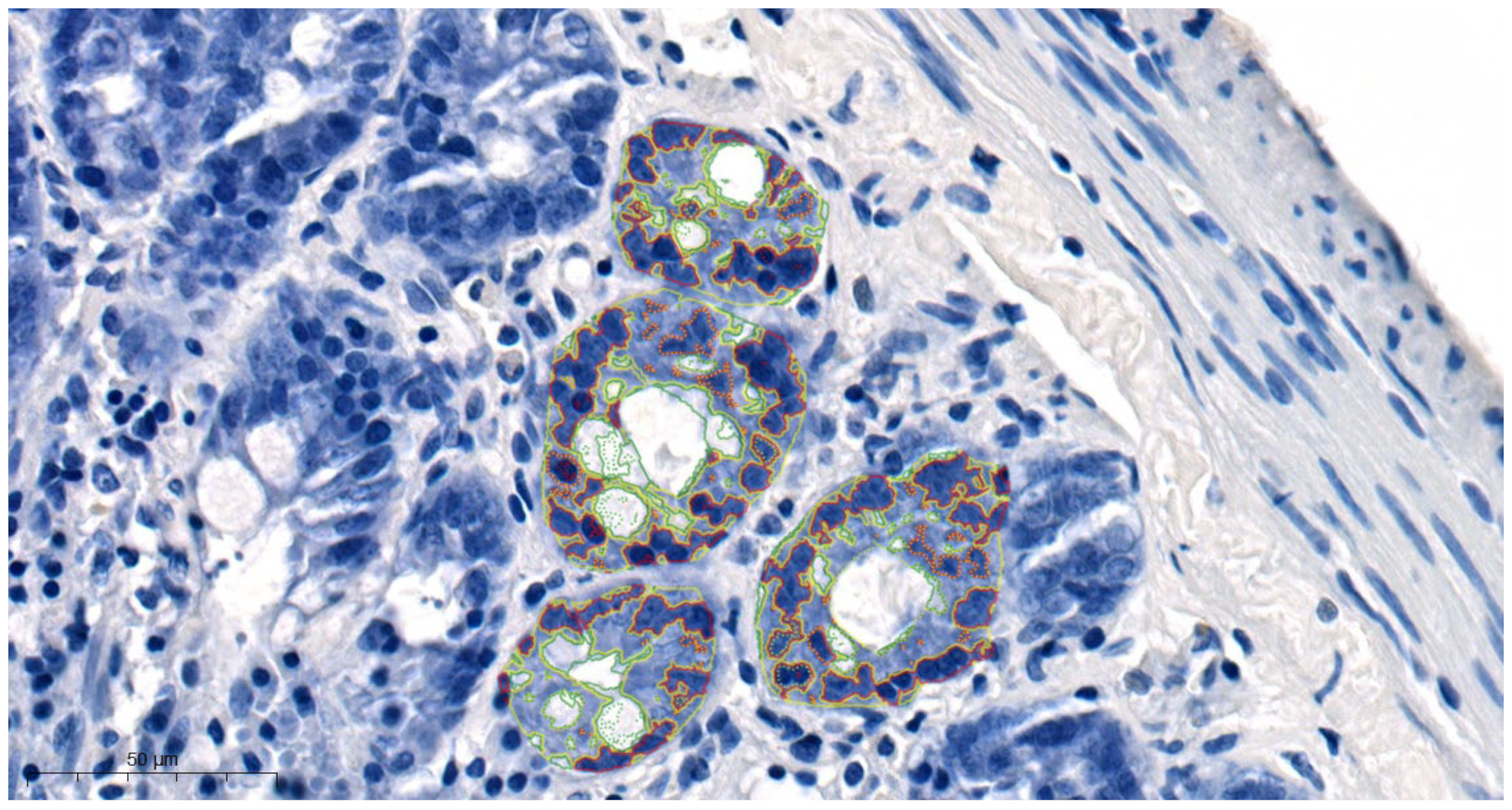"This rectangular image, likely a microscopic close-up view of various small cell structures, displays a complex array of colors and shapes. The top and bottom sides of the image are twice as long as the left and right sides. The photograph primarily features an assortment of blue hues ranging from dark blue to pale blue and blue-gray, interspersed with spots of white. The top left corner is solid white, and within the clear and white cell structures, you can see the background. The gray substance that covers much of the image is dotted with multiple blue and white spots. At the center, four circular structures with green borders contain darker blue circles, each with red and green borders, and light blue interiors. The centers of these circles are white, adding to the intricate and colorful detailing. The scene resembles a scientific sample under a microscope, with various round elements highlighted in green, and a detailed pattern akin to the back of a tortoise shell, but more abstract and cellular in nature."